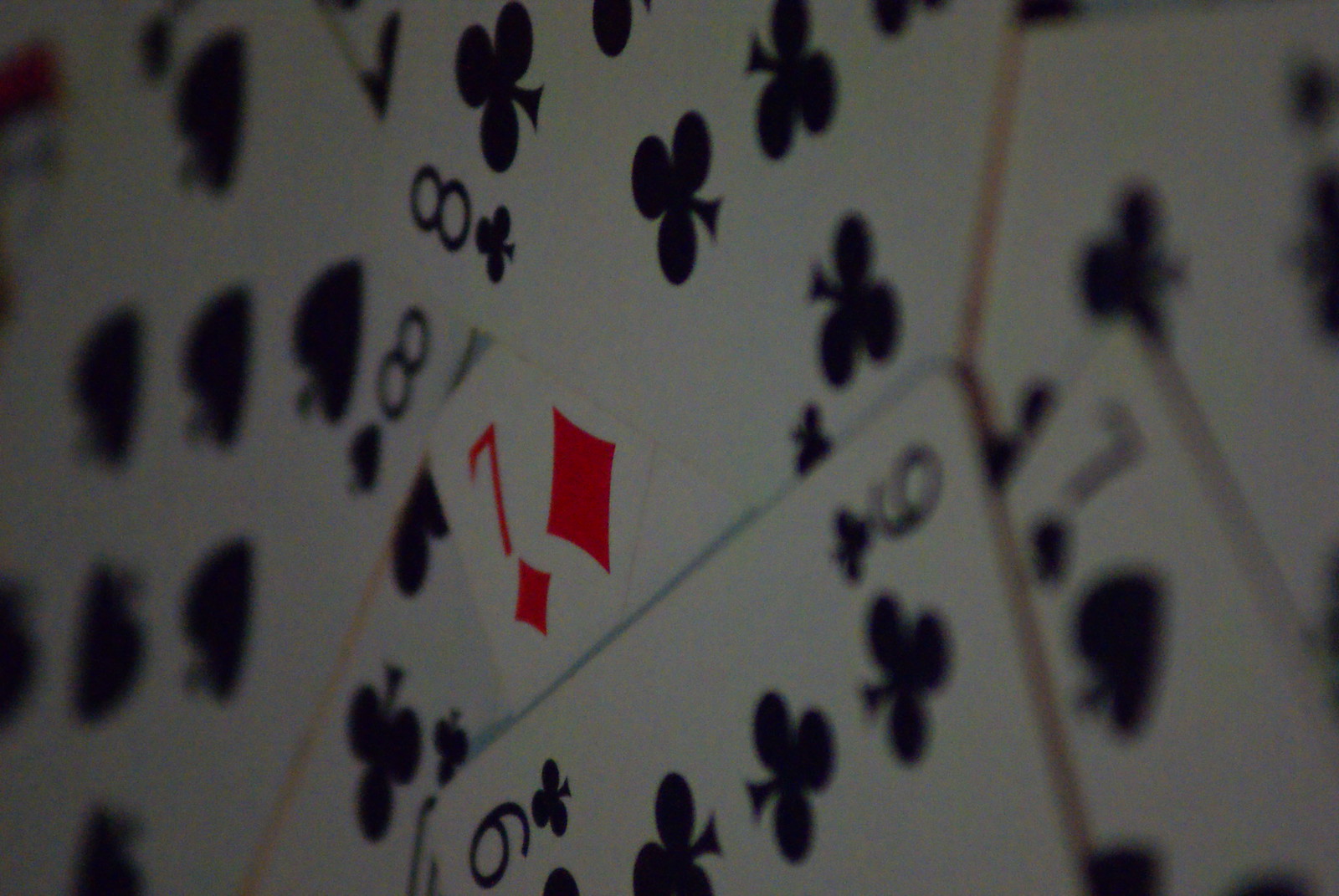In the image, a variety of playing cards are scattered in a slightly disorganized manner. Dominating the composition is a clearly visible Seven of Diamonds, prominently positioned with its top left corner displaying the red number seven and the red diamond icon. Adjacent to it is a slightly out-of-focus Eight of Spades, its black spade symbol somewhat blurred but discernible. Lying diagonally across the Seven of Diamonds is an Eight of Clubs, aligning at a different angle than the surrounding cards. To the right, partially obscured, is a Nine of Clubs, again with its details slightly fuzzy. Beyond this, another indistinct card, the Seven of Spades, appears on the right side of the image, further contributing to the theme of partial blurriness. Intermixed among these cards are more undetermined cards presenting faint patterns, mostly comprising black spades. In this cluster of primarily black-suited cards, the vibrant red of the Seven of Diamonds stands out strikingly against the otherwise monochromatic palette.